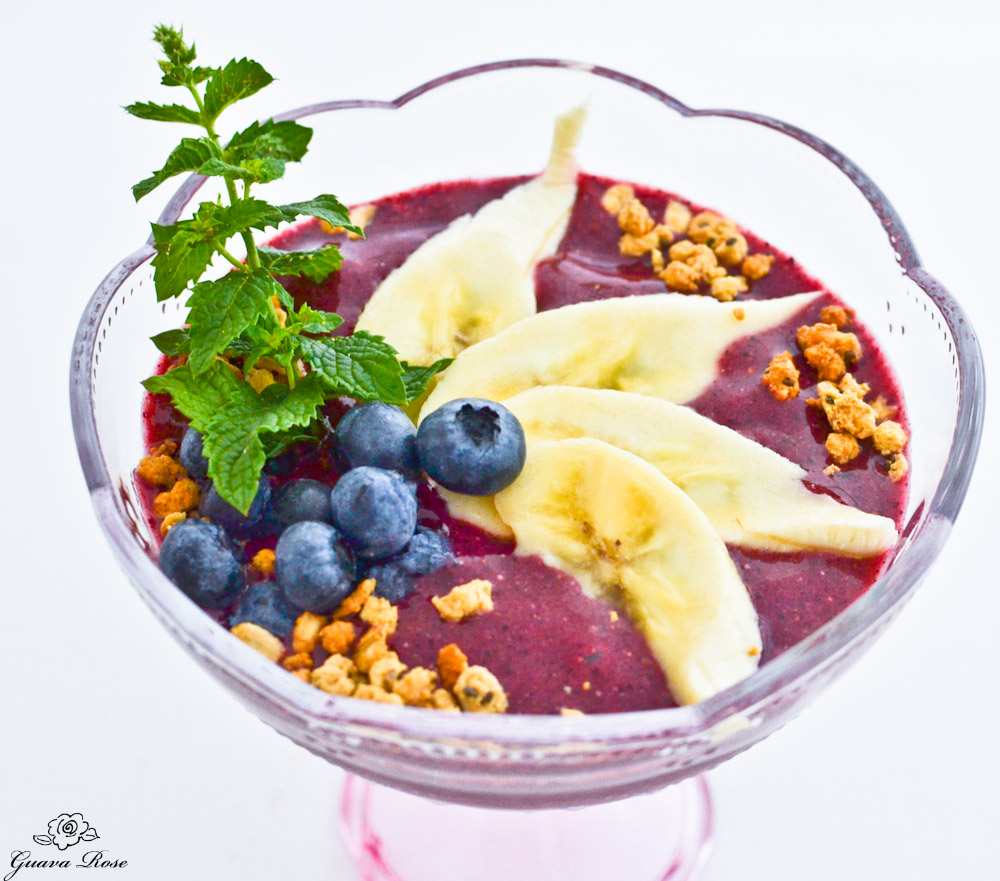The image showcases a stunning artisanal yogurt presented in a tinted purple glass bowl with a pinkish stem. The background is a clean, grey tone, making the colorful dish pop. A small logo featuring the name "Guava Rose" and a rose outline sits in the bottom left corner. Inside the elegant glass bowl, a velvety base of either red or maroon yogurt is beautifully adorned with artistically arranged banana slices fanning out on the right and a scatter of plump blueberries on the left. The dish is further enhanced with crumbles of granola sprinkled on both sides and garnished with a fresh mint leaf. The composition suggests this is an image from a food blog or social media page dedicated to exquisite culinary creations.